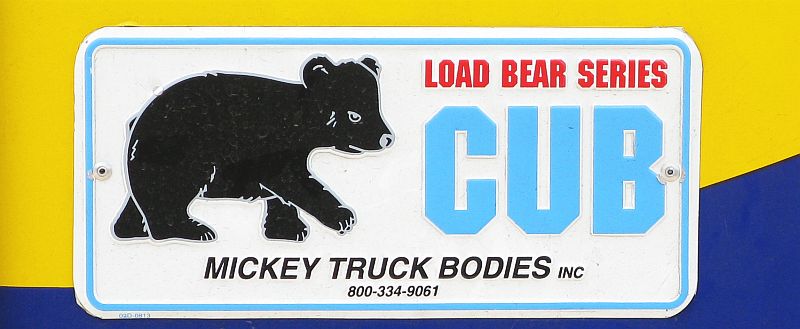The image features a decorative license plate set against a background that is yellow on the top and dark blue on the bottom. The dark blue area starts as a thin strip on the left and expands upward as it moves to the right, covering less space than the yellow. The license plate itself is primarily white with a light blue outline and is attached with screws that are visible on both sides.

Dominating the left side of the license plate is an icon or caricature of a bear cub, depicted in brown or black with white detailing, facing to the right. In the top right corner of the license plate, "Load Bear Series" is written in red letters, and below it, "Cub" is prominently displayed in light blue. Along the bottom, "Mickey Truck Bodies Incorporated" is printed in black, followed by a phone number, "800-334-9061."